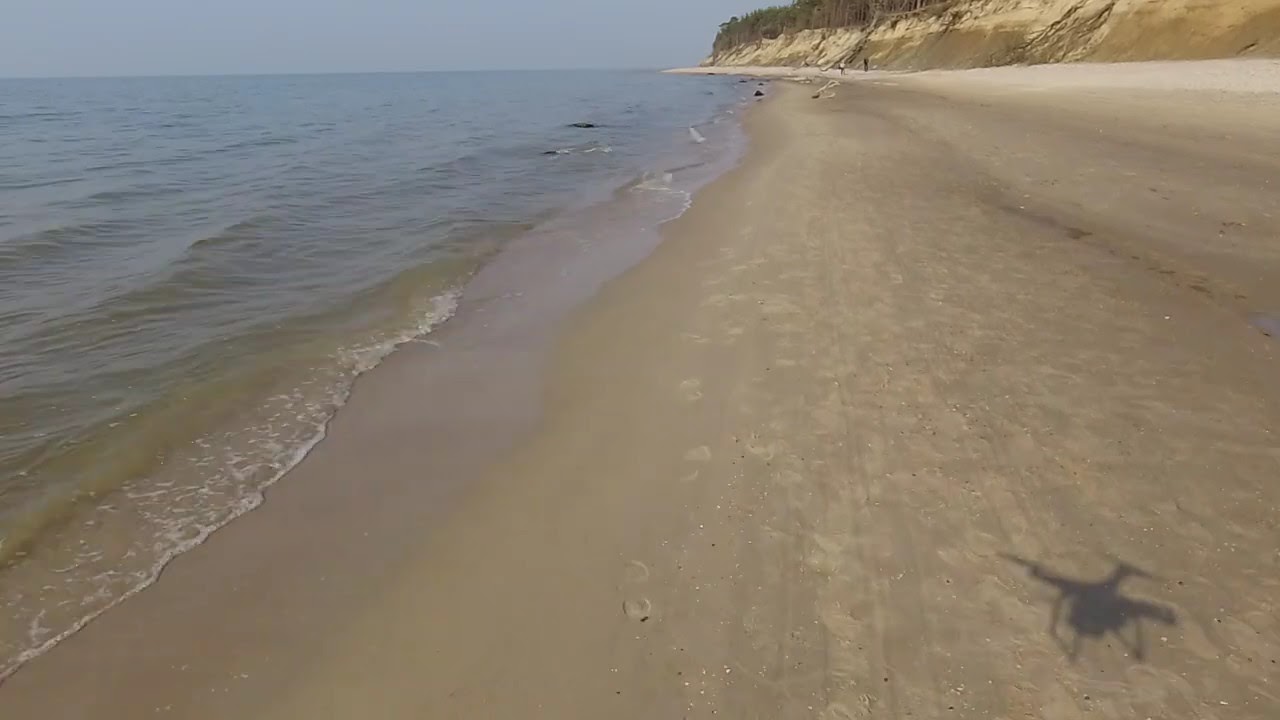This image captures a picturesque beach scene with distinct elements and vibrant colors. The beach spans the right half of the image, characterized by its tan sand which varies in shade due to wetness. Footsteps and tracks are visible on the sand, adding texture and signs of recent activity. On the left side, the ocean waves, bordered by white foamy edges, roll up onto the shore, showcasing a blend of greenish and dark blue hues. The bottom right corner prominently features the shadow of a drone, hinting at an aerial perspective. In the distance, sandy cliffs rise into the sky, darkened in places presumably due to moisture, and topped with a sparse cover of green foliage. The clear blue sky arcs over the entire scene, emphasizing the natural and serene beauty of the landscape. Two distant figures can be seen, adding a sense of scale and life to the otherwise tranquil setting. This photo, likely taken from a drone, offers a comprehensive view of a coastal area blending land, sea, and sky.